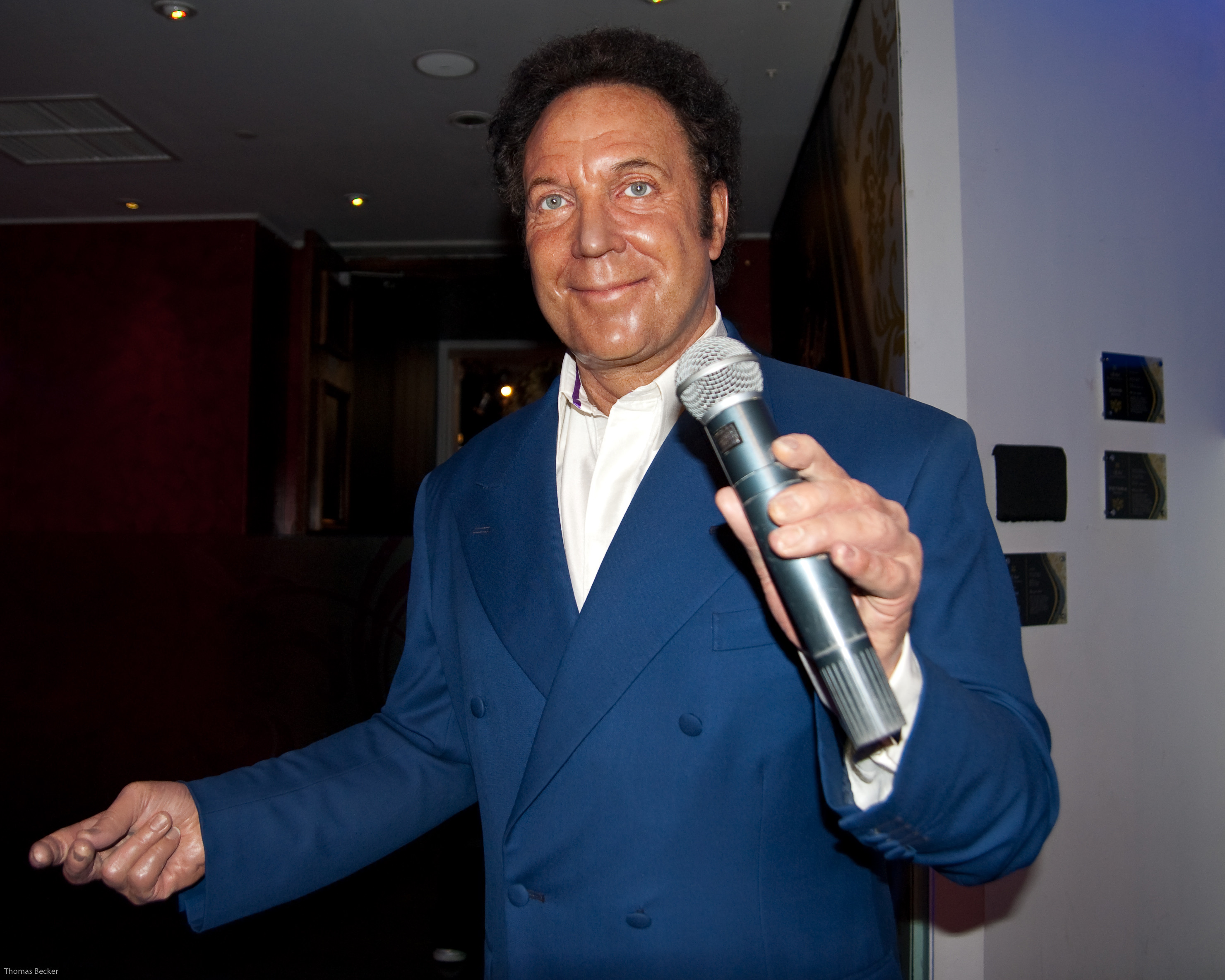This detailed image captures a remarkably lifelike wax figure of the iconic musician and vocalist Tom Jones, likely showcased at Madame Tussauds. The figure, dressed in a deep blue double-breasted sport jacket with two rows of buttons, exudes style with a white open-collar sport shirt underneath. He holds a wireless microphone in his left hand, its silver bulb gleaming, while his right hand appears poised as though snapping his fingers. With short curly brown hair and bluish-gray eyes, the figure offers a closed-mouth smile that brings definition to his cheeks. Tom Jones, depicted younger, perhaps in his 30s or 40s, stands in a dimly lit entryway, possibly of a theater or convention center, with a light gray wall and metal plaques visible to the right. The background features a dark, recessed foyer illuminated by miniature ceiling spotlights, which focus on the figure, making it the radiant centerpiece of the scene.